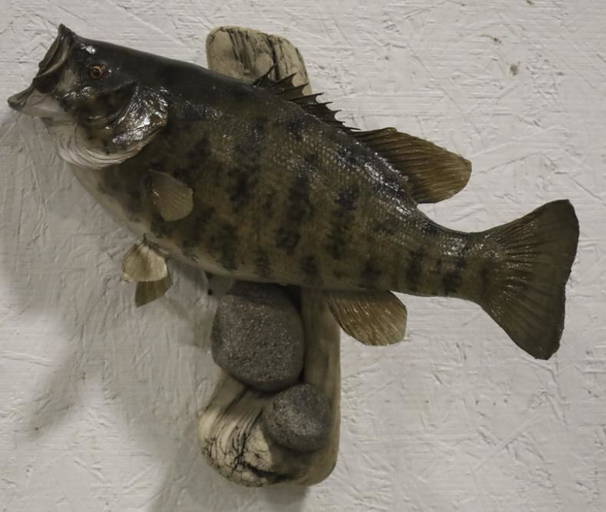The image is a square close-up of a dark brown fish with black spots, mounted with its mouth wide open, facing the upper left corner of the frame. The fish appears to have a glossy, protective coating, and its beaded black eye, encircled with gold, stands out. The underside of the mouth and body are light gray. The fish is pinned perpendicularly to a vertically aligned wooden log or stump, which sits against a white, textured wall resembling painted plywood. Two circular rocks, one brown and one grayish-purple, rest on the log beneath the fish. The fish casts a shadow to the left, indicating a light source from the top right.